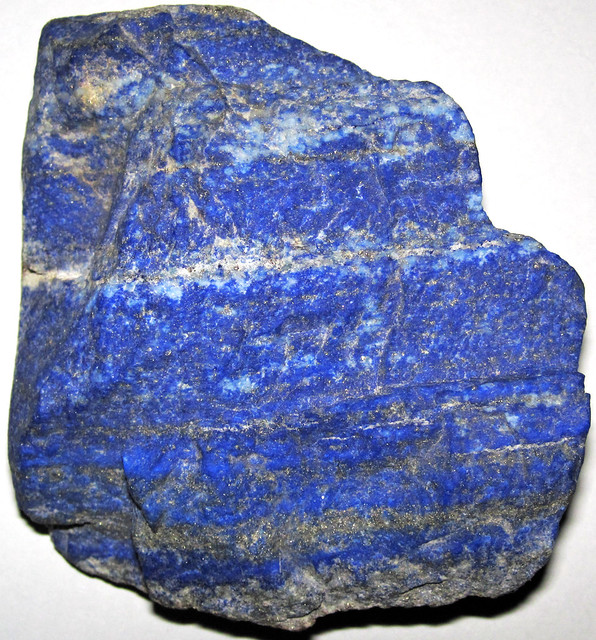This image is a close-up photograph of a semi-precious stone, lapis lazuli, displayed on a plain white background. The stone dominates the frame, appearing mostly flat and somewhat rectangular, though the top right corner is irregular and wavy. The lapis lazuli showcases a vibrant, royal blue color, marbled with specks and horizontal veins of gray and white. The varying shades of gray create a gradient effect, darkening towards the bottom of the stone with a striking lighter gray band running through the center. The texture appears bumpy, suggesting it is in its uncut form. The image perspective, likely a bird’s eye view, emphasizes the intricate details and coloration, making it a captivating specimen often used in jewelry.